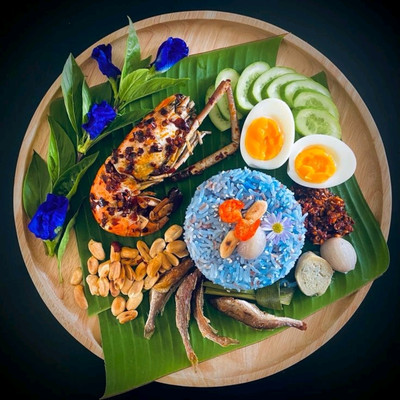The photograph displays a top-down view of a culinary arrangement on a decorative circular wooden plate set against a black background. Centered on the large banana leaf, which serves as a bed, is a diverse assortment of food items. The focal point is a succulent, chili-flake-crusted lobster. Surrounding the lobster is a mound of vibrant light blue rice, adorned with a blue flower, peanuts, and chili. Flanking the rice are four small dried sardines. Adjacent to these elements, you find cucumber slices and two halves of a hard-boiled egg. A small portion of red chili paste and some garlic cloves are also present. Bright blue flowers and a herb garnishing decorate the top-left of the plate, enhancing the visual appeal of the presentation.